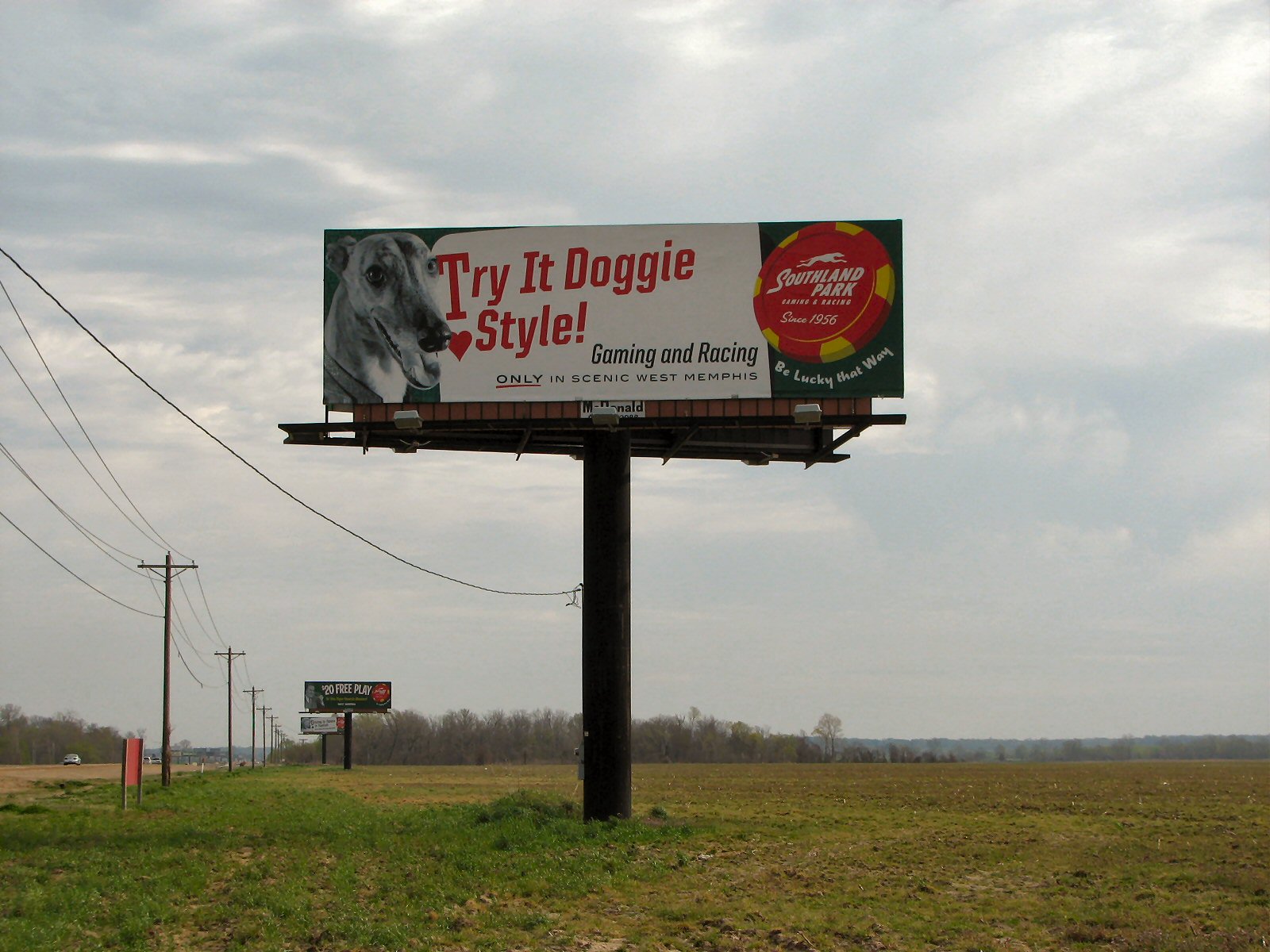In this image, a wide expanse of open farmland stretches out, bordered on the left by a road. A series of telegraph wires traverse the scene horizontally. Prominently in the foreground, a large sign is mounted on a post. The sign is predominantly white with bold red eccentric capital letters that read, "TRY IT DOGGY STYLE – GAMING AND RACING." To the right of this message, the sign denotes the name of a park, though the specifics are partially obscured in the image. The backdrop features a blue sky mottled with a thick layer of blurry, cloudy formations, suggesting an overcast day without active rainfall. A smaller red sign can be seen by the roadside, adding a touch of additional color to the landscape.